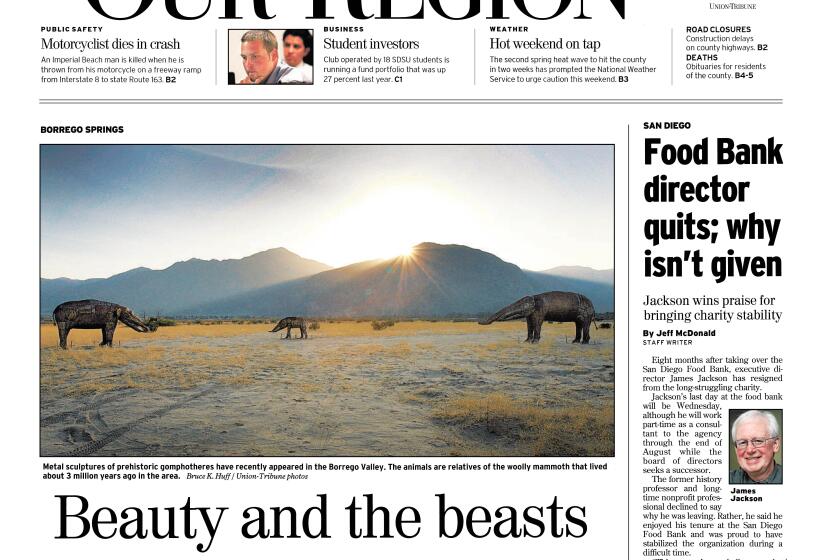The front page of this newspaper prominently features a captivating photograph titled "Beauty and the Beast." The center of attention is a stunning display of metal sculptures depicting prehistoric Gamboa creatures, distant relatives of the woolly mammoths that roamed the Baringo Valley approximately three million years ago. These sculptures are strikingly realistic, encapsulating both familiar and otherworldly qualities.

In the background, the sun bathes the scene in a warm glow as it either rises or sets behind a range of majestic mountains. The landscape is predominantly desert-like, interspersed with patches of yellow grass. A clear blue sky, accentuated by a radiant ring of sunlight, adds to the enchanting atmosphere captured by photographer Bruce K. Huff of the Unison Tribune.

To the right of the main image, another article announces the resignation of the local food bank director. The headline reads, "Food Bank Director Quits," with a subheading questioning the reasoning behind the departure. Accompanying this news is a photograph of James Jackson, presumably the outgoing director, offering a glimpse into the content that continues below the fold.